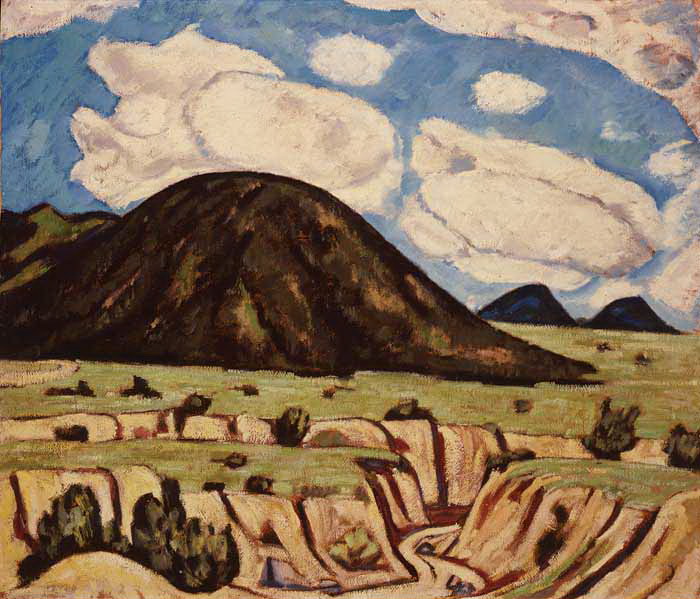This detailed painting captures a serene landscape, likely created using watercolors or colored pencils. The sky is a vivid blue with varying streaks and shades, punctuated by thick, bulky clouds that have gray patches, giving them an almost potato-like, substantial appearance. The backdrop showcases several hills and mountains: two dark blue ones in the far distance, and a large dark brown mountain with patches of green grasses covering it. The grassy field in the foreground is a light mint green, contrasting beautifully with the darker hues of the mountains. Cutting through this verdant expanse are dry, sandy-looking riverbeds where water once flowed, now mostly dry. This tranquil scene is completed with details of bushes and rocks scattered across the landscape, devoid of any human presence or textual elements.